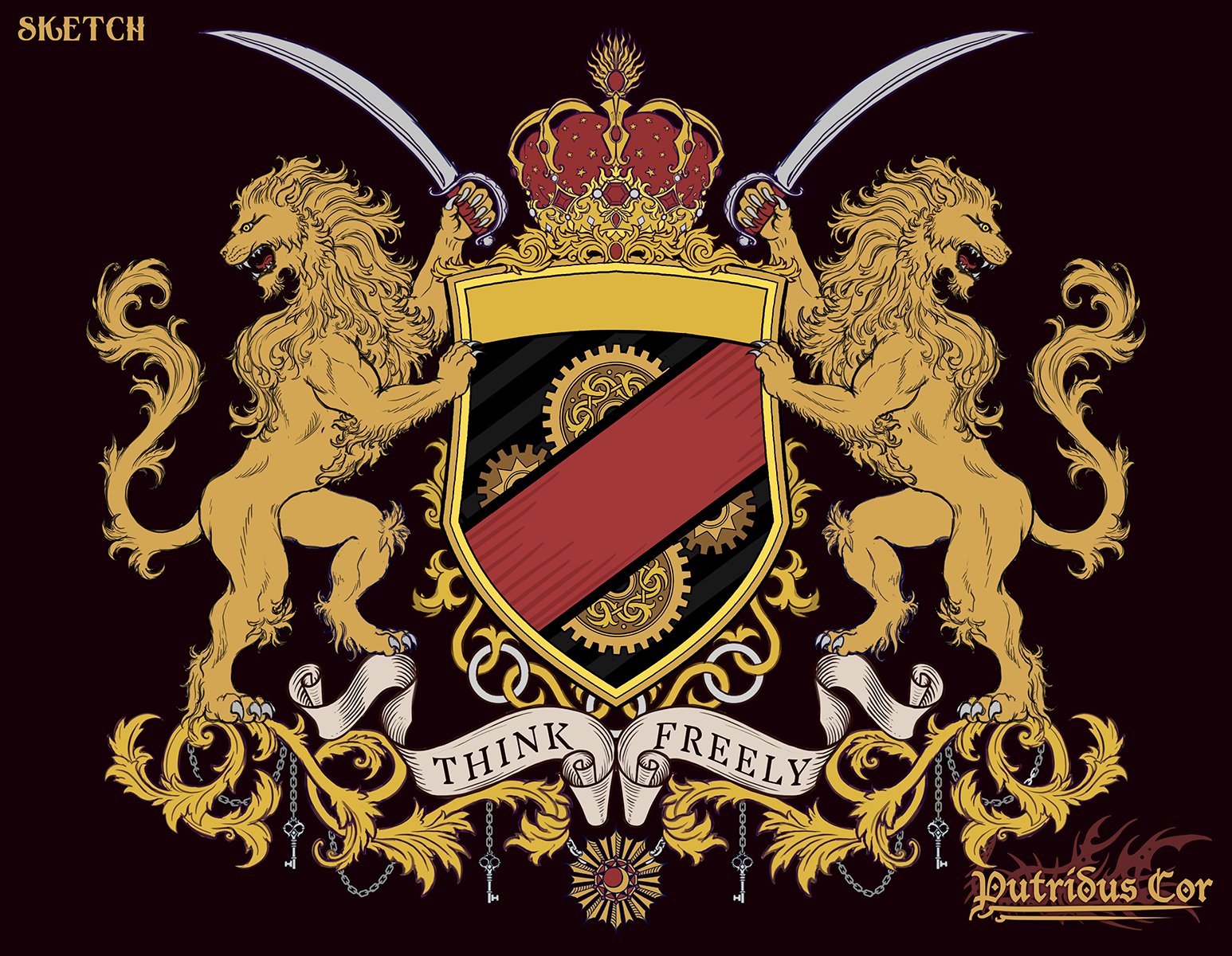This horizontal, rectangular image showcases a detailed coat of arms against a black background. In the upper left corner, the word "SKETCH" is clearly written in gold letters, while in the lower right corner, the phrase "PUTRIDISCORE" appears, underlined by two lines, indicating the name of the organization. Central to the coat of arms are two very muscular lions, each standing on either side while holding swords with clawed hands. Their faces are turned away from each other, pointing toward the left and right edges of the image.

Dominating the center is a crest featuring a bold gold stripe along the top and a red bar encompassing the rest. Above this central shield sits an elaborate golden crown lined with red. Beneath the crest are white scrolls of paper with the phrase "THINK FREELY" inscribed in black ink. 

The primary colors of the emblem are yellow and red, decorating various elements like the crown and scrolls. Swirling designs and what appear to be keys can be seen at the feet of the lions, adding intricate details to the composition.